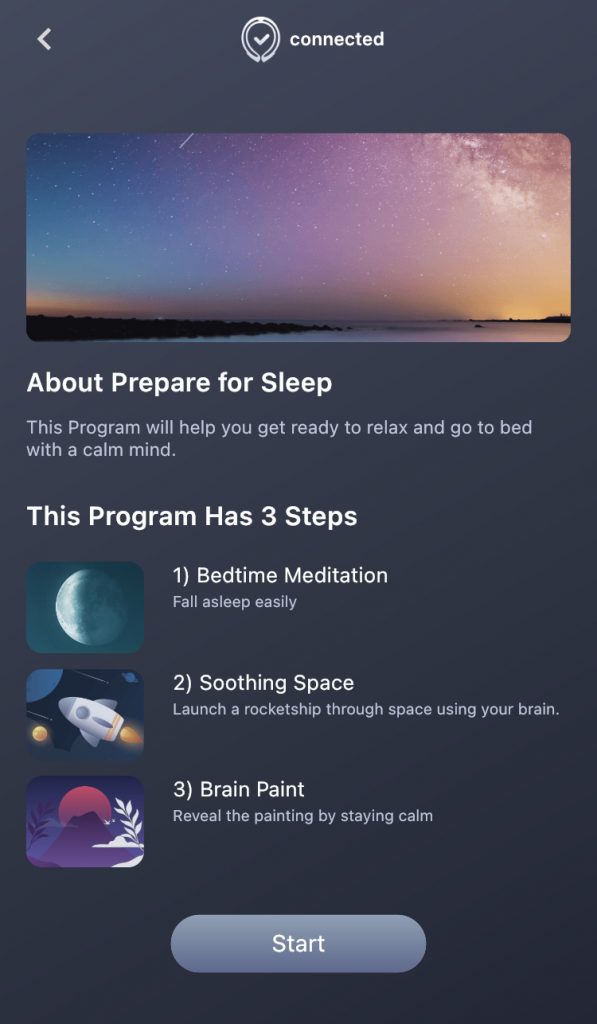This image, likely from a sleep app, showcases a well-organized interface set against a dark, chocolatey-gray background. At the top, a white checkmark icon within a location symbol is accompanied by a back arrow, all beneath the lowercase white text reading "connected." Below this header is a serene, twilight landscape photo, featuring a lake bordered by low-rise, silhouetted trees. The sky transitions from deep blue at the top to a blend of purple and orange hues above the horizon.

Beneath the image, the text "About: Prepare for Sleep" introduces a program designed to help users relax and prepare for bedtime with a calm mind. The description mentions that the program includes three steps. To the lower left of the text, three pictures are stacked vertically, each representing one of the steps.

- The first step features a moon icon labeled "Bedtime Meditation," with a subtitle encouraging users to "fall asleep easily."
- The second step displays a cartoon rocket ship labeled "Soothing Space," suggesting a journey through space using one's imagination.
- The third step, titled "Brain Paint," is depicted with an artistic image involving a man in white flanked by foliage and a red moon, with instructions to "reveal the painting by staying calm."

Each step is designed to guide users through a soothing experience aimed at promoting restful sleep.